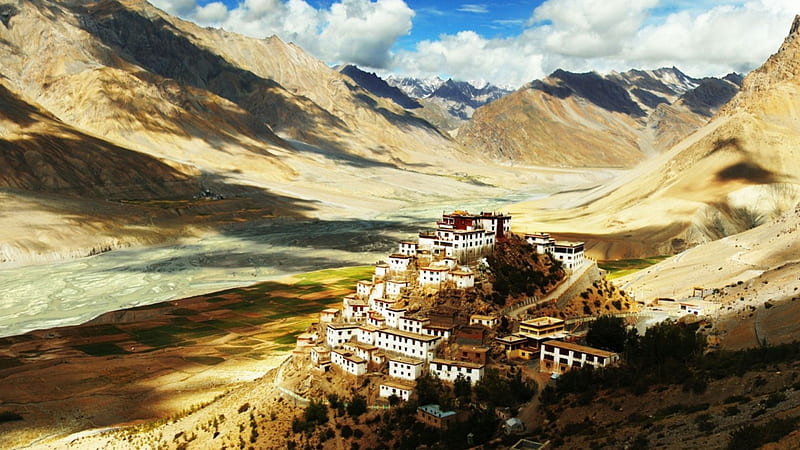The image depicts an isolated civilization, likely historical, built entirely on the slopes of a single mountain amidst a desert landscape. The mountain's winding road is lined with numerous white buildings, each topped with flat brown roofs, giving a uniform appearance regardless of their size. Surrounding the settlement are towering tan mountains with steep cliffs, creating a dramatic backdrop. The valley below features sparse greenery, including some brown plants, trees, and patches of grass. Despite the arid predominance, splashes of green vegetation can be seen near the rock formations. The sky above is a striking blue, dotted with puffy white clouds, suggesting a beautiful but remote and challenging environment. The absence of visible people, text, or modern amenities like grocery stores, coupled with the potential presence of snow-covered distant mountains, adds to the sense of isolation and antiquity. This hidden city, captured from a distant vantage point, evokes a sense of mystery about its past and present inhabitants.